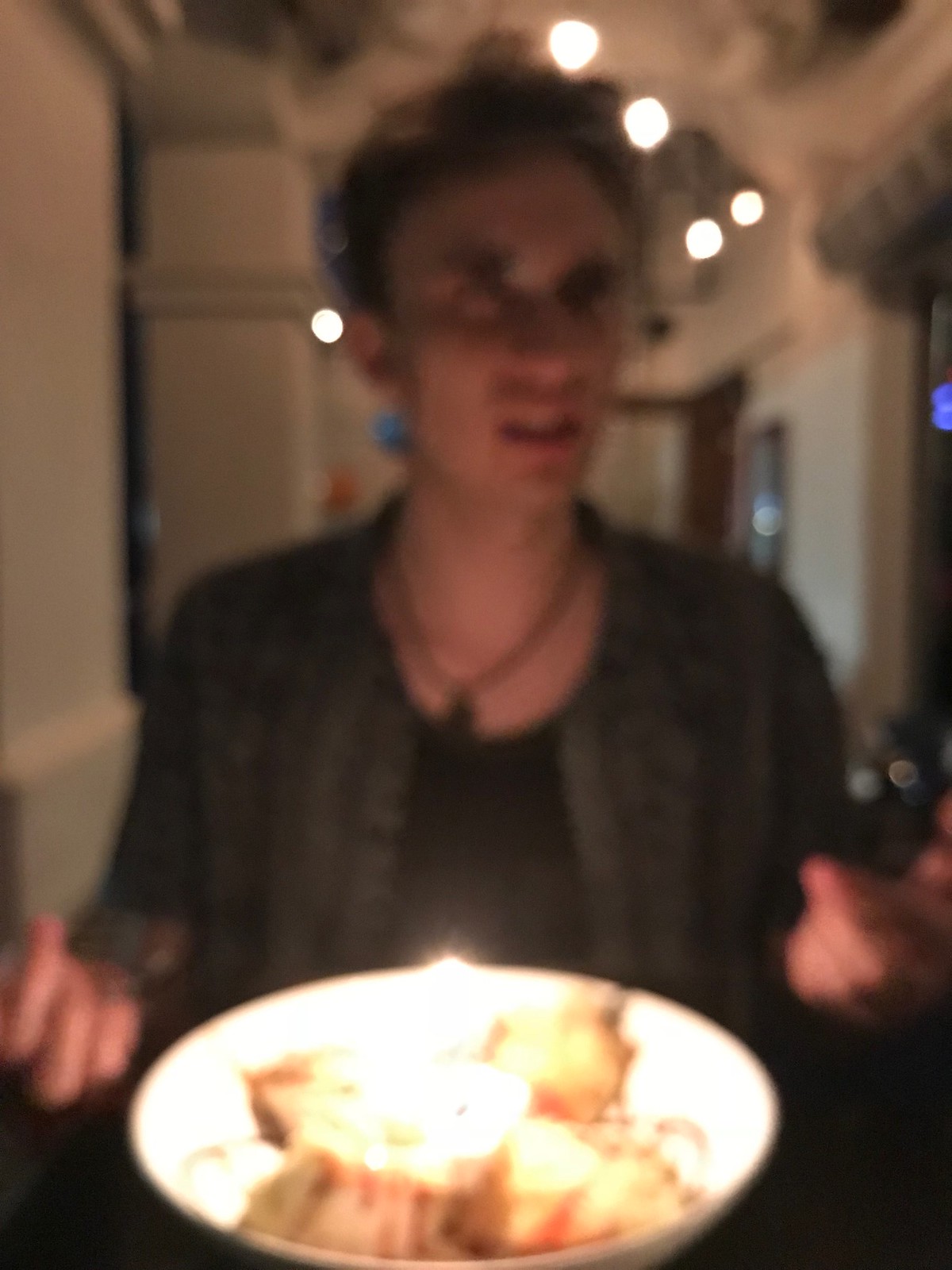In this image, a man is positioned either sitting or standing in front of a table or a bar-height counter, engaged in an intense conversation, accentuated by his animated hand gestures. He wears a black shirt layered with a gray jacket, and around his neck dangles a small necklace on a string. His demeanor expresses displeasure as he directs his gaze toward someone off-camera. 

In front of him, there is an oversized white bowl filled with what appears to be a freshly-prepared meal. Ambient light reflections create a halo effect around his head, adding a unique visual interest to the scene. The background suggests a restaurant setting, with visible cream-colored walls, long windows, and several pillars. A glass door can be seen off to the side. The subtle lighting adds warmth to the atmosphere, and a soft yellow glow appears to be emanating from or reflecting off the food in the bowl, possibly from a nearby candle.